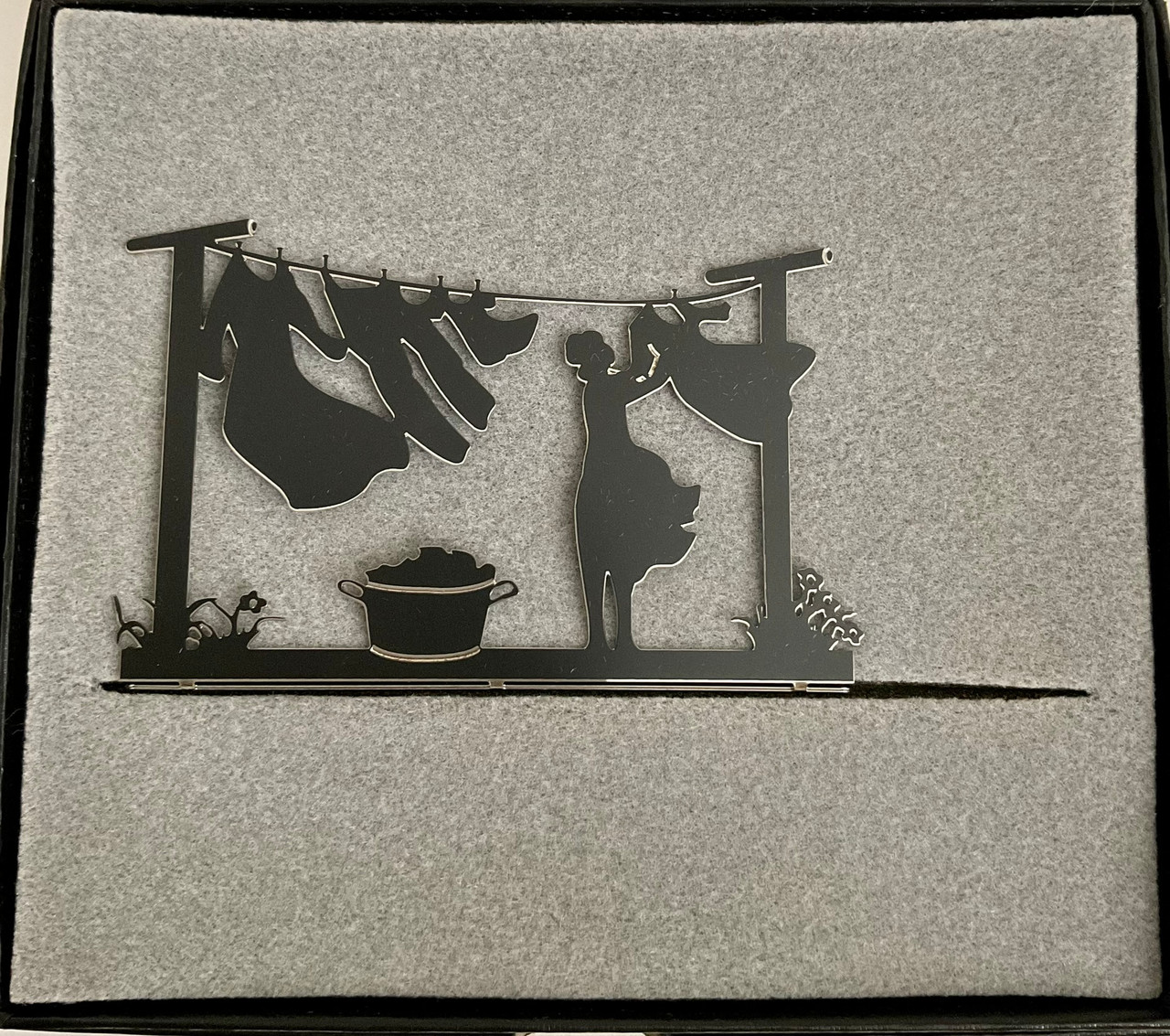This intricate piece of metal art captures a serene moment of a woman hanging laundry. The black metal cutout, meticulously crafted and displayed on a gray felt background within a black frame, illustrates her task with fine detail. The woman, wearing a dress that billows in the wind, reaches up to hang another dress on a metal clothesline suspended between two T-shaped poles. Already on the line are a flowing dress, a pair of pants, and a small child's dress, each secured with two clothespins. At her feet, a wicker basket brims with laundry. Adorning the bases of the clothesline poles are delicate cutouts of flowers and grass, emphasizing the outdoor setting. The dynamic angles of the clothing and the woman's dress beautifully depict a breezy day, all thoughtfully etched in metal. This impressive work is both detailed and evocative, showcasing the artistry and attention to detail involved in its creation.